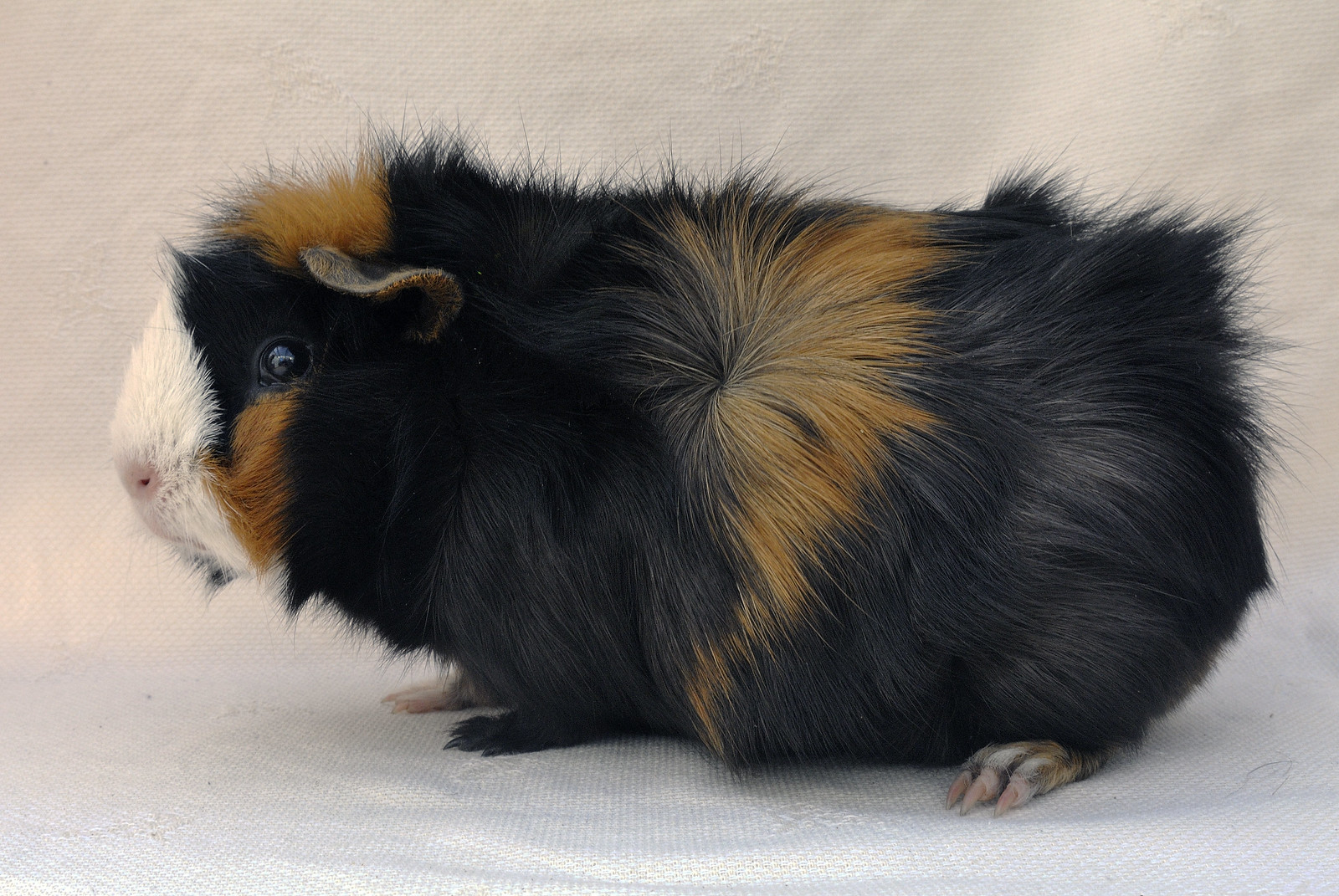This is a close-up photograph of a juvenile guinea pig, positioned on a white background and standing on a white surface, possibly a towel. The guinea pig is facing to the left and displays a calico pattern, predominantly black with bright orange patches. Specifically, there's an orange stripe in the middle of its body, an orange spot on top of its head, and an orange spot below the left eye on its left cheek. The guinea pig's nose and muzzle area are white, with the nose being pink. Its right front foot is white, the left front foot is black, and the left rear foot is mostly white with some orange and black spots. The guinea pig has distinctive puffy cheeks, a hallmark of its rodent-like appearance, and displays a healthy, somewhat untamed coat, with fur pointing in various directions. It has a single visible black eye and one ear showing.